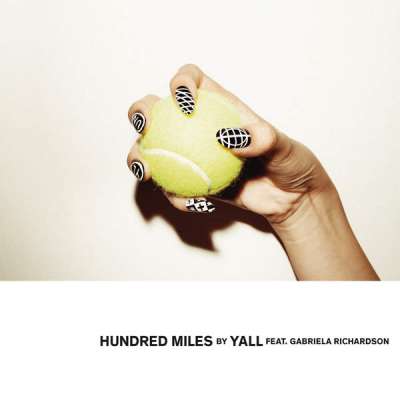The image displays a detailed close-up of a Caucasian woman's hand with long, pointy fingernails, painted black with intricate white patterns. Each nail carries a unique design, featuring crosshatch and spider-web-like patterns. The hand is tightly clasping a pastel lime-colored tennis ball, compressing it so much that the white lines on the ball are visible. The background of the photo is a cream or off-white color. At the bottom of the image, black text reads "100 Miles by Y'al Featuring Gabrielle Richardson," suggesting that this could be an album cover for a music single or LP.